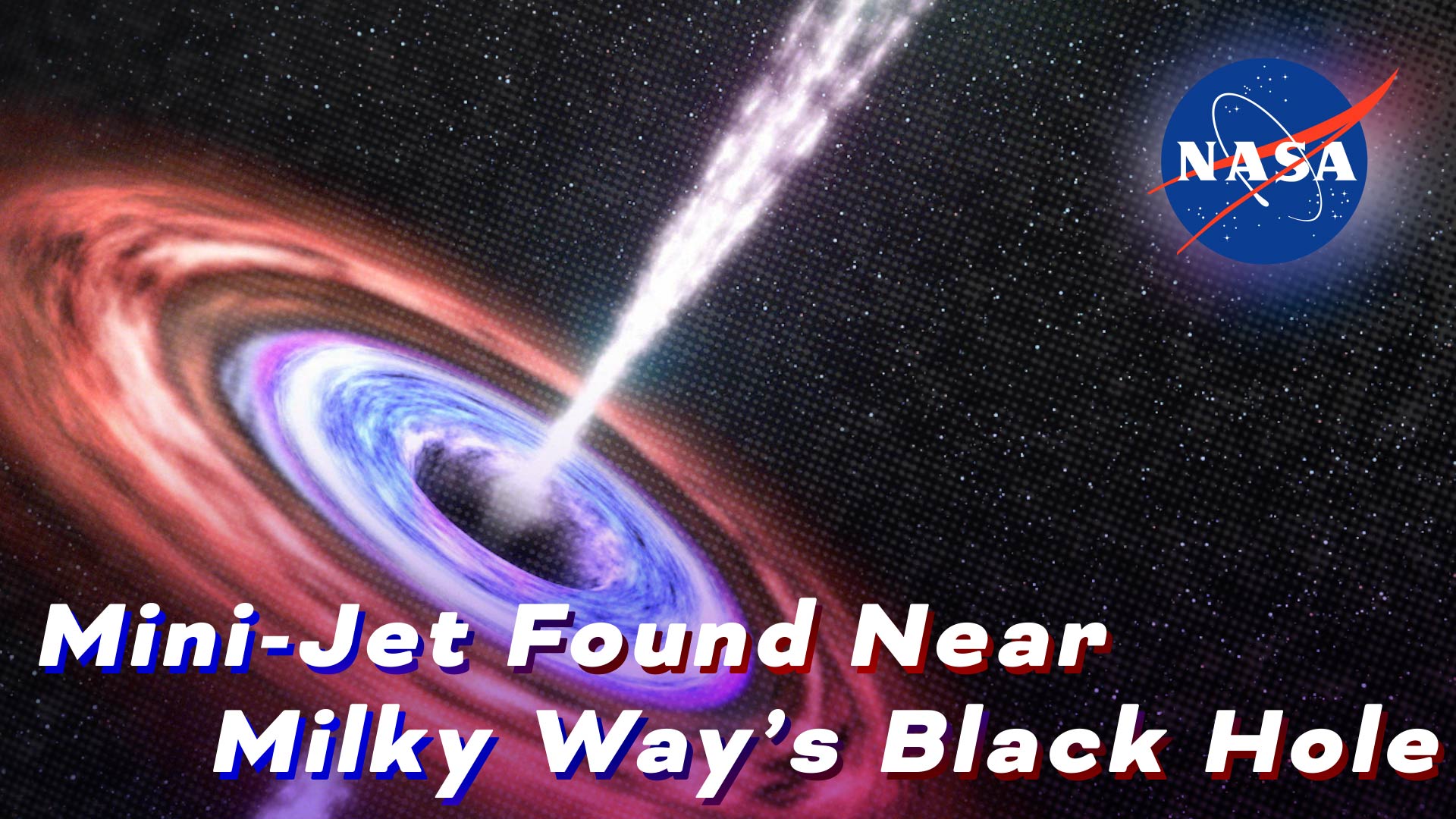The NASA image displays the vastness of deep space against a black backdrop speckled with white stars. Prominently positioned in the upper right corner is the iconic NASA "meatball" logo, a blue circle with the white letters NASA, accented by a red orbit-style streak and surrounding elements. Dominating the left side, from the upper left to the bottom left, is a vibrant artist’s depiction of a black hole located in the Milky Way. This phenomenon features a striking series of concentric rings: the innermost rings are a stunning mix of blue, white, and purple hues, transitioning outward to layers of dark red, light red, and orange. Piercing through the center of these rings is a powerful white beam, illustrating a mini jet. Below this vivid illustration, large white text reads, "Mini Jet Found Near Milky Way's Black Hole," highlighting the subject of the graphic. The meticulous details of the black hole, combined with the surrounding cosmic elements and descriptive labeling, create an informative and eye-catching space graphic.